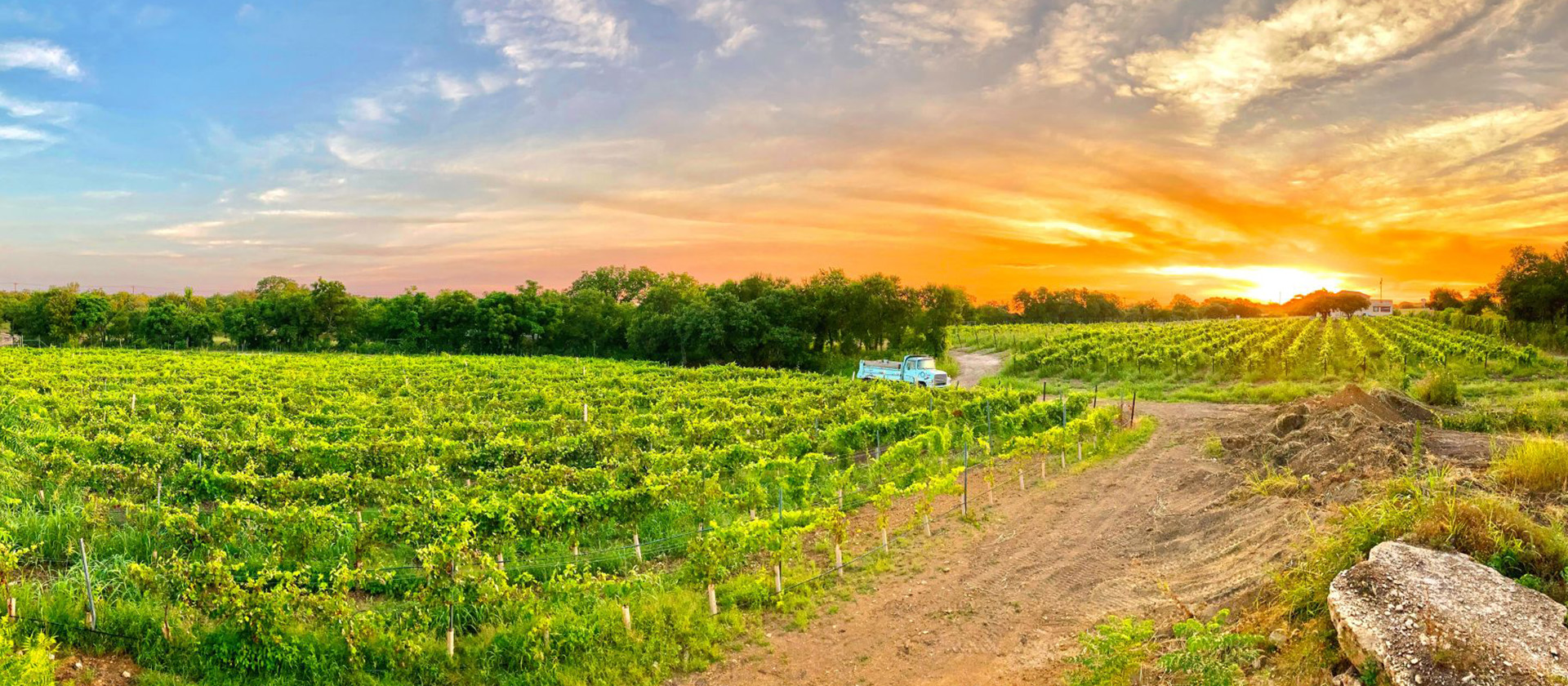The image depicts a tranquil farm scene at sunset, with expansive green farmland in both the foreground and background. A brown dirt road meanders through the landscape, where a light blue pickup truck is seen traveling in the distance. The sky occupies the upper third of the image, ablaze with the vibrant hues of the setting sun, transitioning from deep orange and yellow to pink, purple, and blue, adorned with striated clouds. Neat rows of vegetation, interspersed with labeling stakes, stretch across the farm, demonstrating meticulous care. In the background, a line of dark green trees marks the horizon, providing a natural border to the cultivated land. A large stone rests in the lower right-hand corner, adding a rustic touch to the serene agricultural vista.